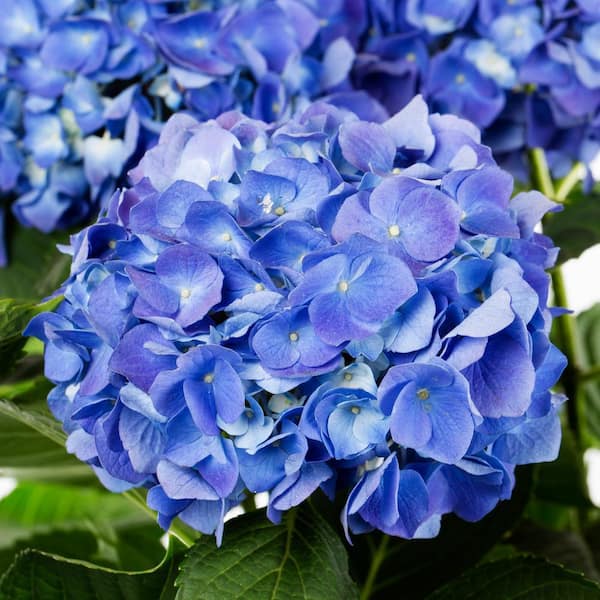A vibrant close-up photograph captures an exquisite blue hydrangea in full bloom, displaying its tightly packed, violet-blue petals that form a rounded and dense cluster. Each blossom is accentuated by small yellow dots at its center, adding a striking contrast to the intense hue of the petals. The green leaves, with their distinct edges and ridges, provide a lush background, revealing visible veins under the bright light that illuminates the scene. Surrounding the focal hydrangea are additional clusters of similarly colored flowers, slightly blurred to emphasize the main bloom, with hints of purplish-pink and light blue tones. The photograph features speckles of white light filtering through, giving the entire image a dynamic and lively appearance.